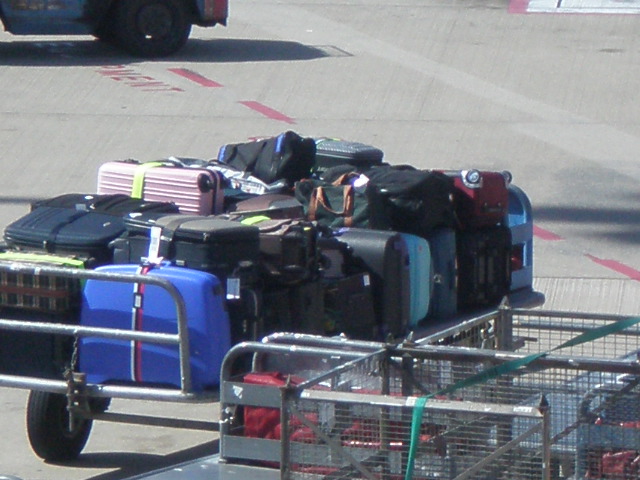The photograph showcases a bustling scene on an airport tarmac, featuring a large metal-framed baggage cart loaded with an array of suitcases. The luggage varies in shape, size, and color—ranging from soft to hard shell types, with bold hues like pink and royal blue, and some secured with baggage straps. The cart, situated centrally, is surrounded by the expanse of the tarmac, marked with red paint lines and indistinct stamped words in the background. Partially visible in the right foreground are additional trailers, featuring wired metal cages secured with green straps, possibly designed for different types of cargo. In the top left corner, the rear wheels and lower side of a truck are just discernible, adding to the airport's busy atmosphere. The image captures the organized chaos of luggage handling, readying myriad pieces for transit.